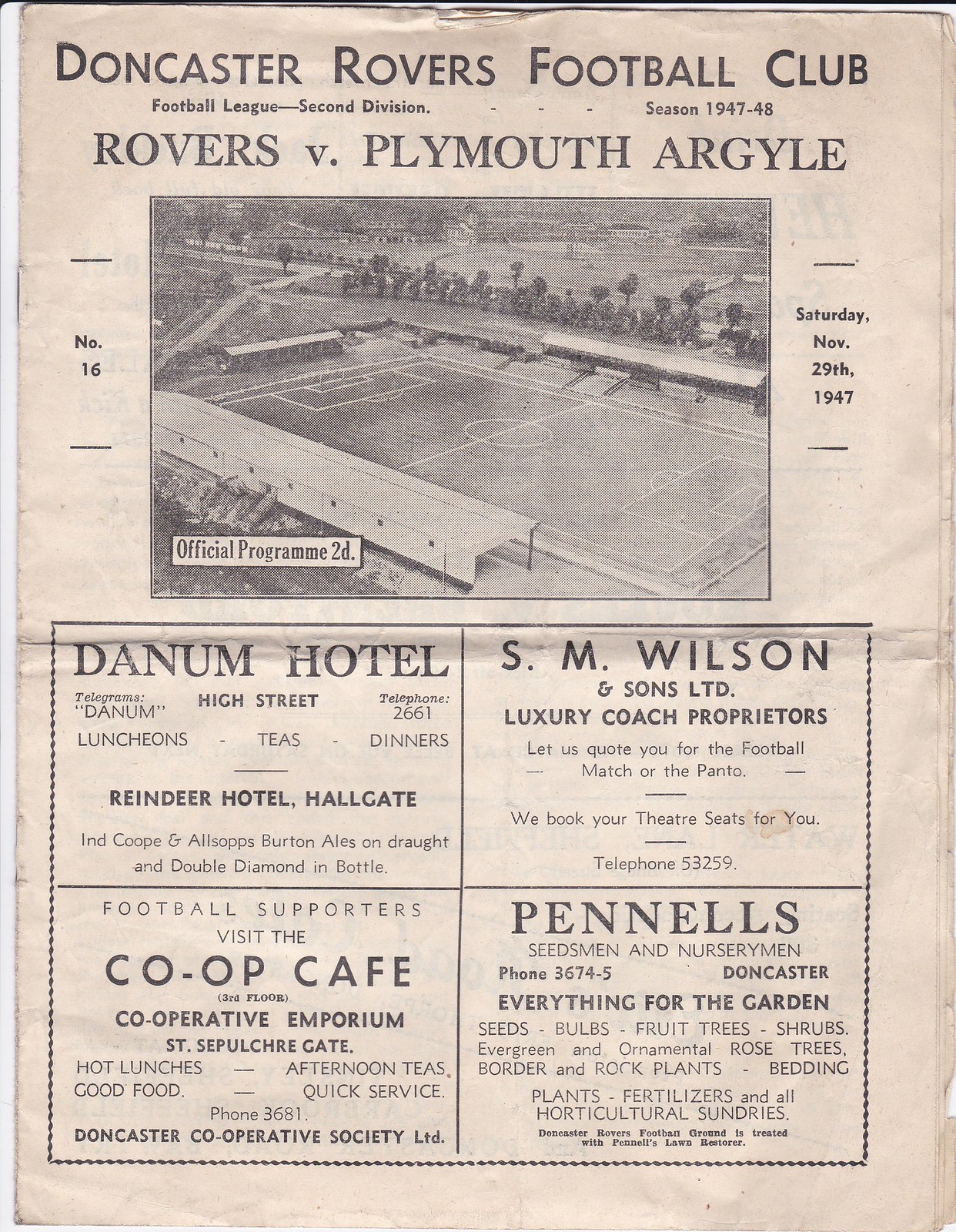This promotional flyer for the Doncaster Rovers Football Club showcases a vintage newspaper or magazine design, resembling parchment paper. The top section boldly reads "Doncaster Rovewells Football Club" with "Football League 2nd Division, Season 1947-48" printed below. Prominently displayed beneath is "Rovers v. Plymouth Argyle", marking the game held on Saturday, November 29, 1947. An aerial, black-and-white photograph of a football stadium, captioned "Official Program 2d," occupies the center. The left side of the image is marked with "number 16", and the right side reiterates the date. The bottom half of the flyer consists of four rectangular advertisements organized in two rows: Denham Hotel (top left), S.M. Wilson (top right), Co-op Cafe (bottom left), and Pennell's Seedsmen and Nurserymen (bottom right). These ads suggest sponsorship for the event. The overall style epitomizes vintage graphic design printing.